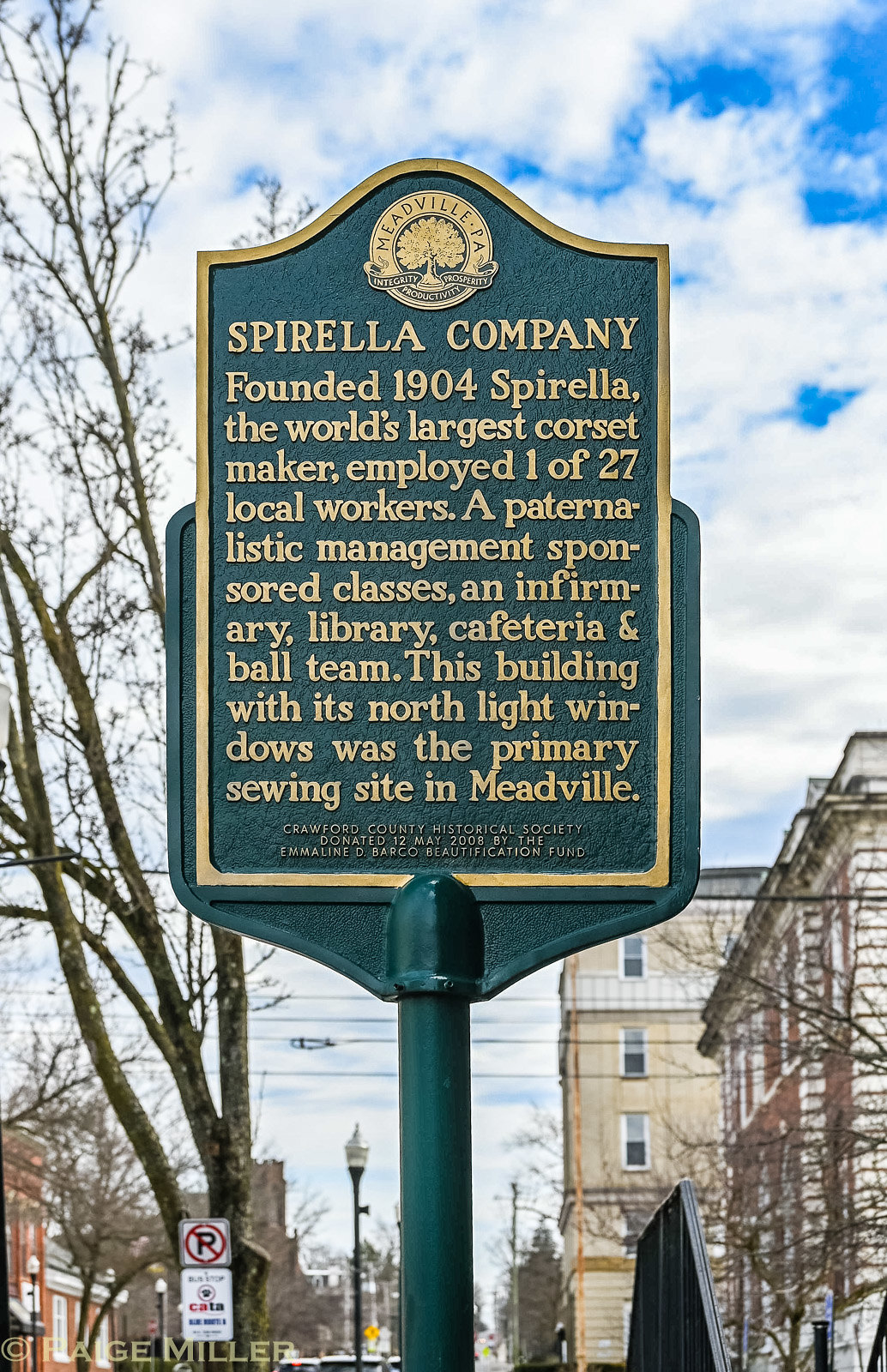In the foreground of the image, there is a prominently positioned informational sign mounted on a green pole with dark green detailing. The sign is bordered in gold and features a shield-like design, topped with a circular logo depicting a fully leafed tree, along with the inscription "Meadville, PA." The text on the sign provides a detailed history of the Spirella Company, established in 1904. This company, once the world's largest corset maker, employed 27 local workers and had a paternalistic management that offered classes, an infirmary, a library, a cafeteria, and sponsored a ball team. It mentions that this building, characterized by its north light windows, was the primary sewing site in Meadville. Surrounding the sign is a scene with several notable elements: a bright blue sky filled with large, white puffy clouds, city buildings on both sides that are older and middle-sized with flat roofs made of yellow and red brick, and a spindly, tall tree devoid of leaves. Additional background details include multiple street signs, such as a no parking sign, streetlamp posts, railings, and the faint tops of some cars. An old-fashioned lighting fixture is also visible behind and to the right of the sign.